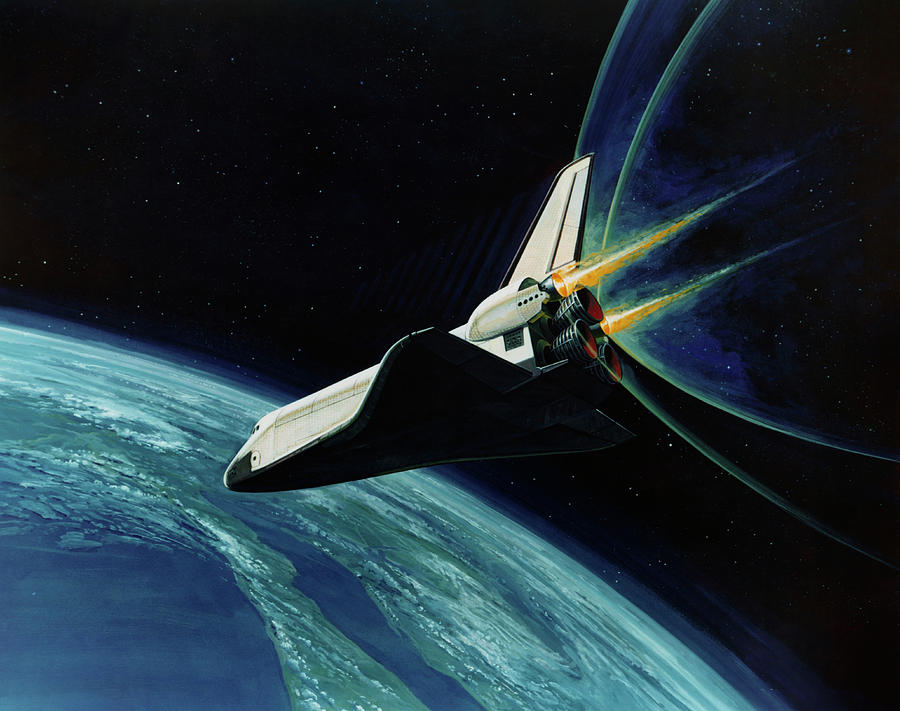This detailed illustration, likely created by painting or AI, showcases a rocket ship zooming towards Earth against the vast blackness of outer space, dotted with faint stars. The central focus is the rocket ship, colored predominantly white with black and rusty, sandy-colored lines. Bright orange fire emanates from its back, alongside peculiar L-shaped loops of green and blue lights that add a surreal touch. The bottom left corner of the image reveals a partial view of Earth, depicting an amalgamation of indistinct, scattered landmasses and turquoise oceans, some shrouded in clouds. The overall scene is vibrant yet slightly offbeat, with elements that blend the realistic and the fantastical.